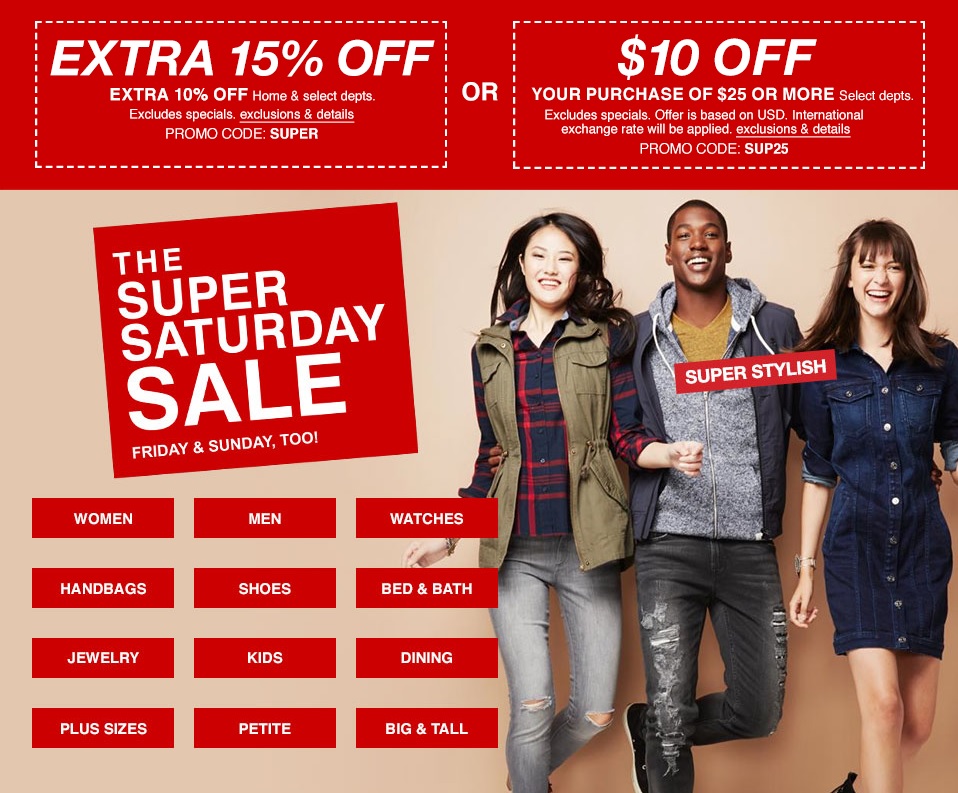This website image showcases a clothing retailer's homepage, prominently displaying a diverse group of models in fashionable attire in the bottom right corner. On the far left, an Asian woman with dark black hair sports a chic outfit: a brown vest over a black top accentuated with red stripes, paired with light blue pants. Standing beside her, a stylish Black man dons a gray vest layered over a dark gray jacket, a bright yellow undershirt, and ripped black pants. Completing the trio is a White woman with brown hair, elegantly dressed in a dark blue denim dress, accessorized with a watch on her right wrist.

To the left of these models are three rows of neatly organized category boxes, aiding in navigation through the website's diverse product offerings. The top row features categories for Women, Men, and Watches; the second row includes Handbags, Shoes, and Bed & Bath; while the third row presents Jewelry, Kids, and Dining options. Ensuring inclusivity, the bottom row highlights specialized sizes including Plus Sizes, Petite, and Big & Tall.